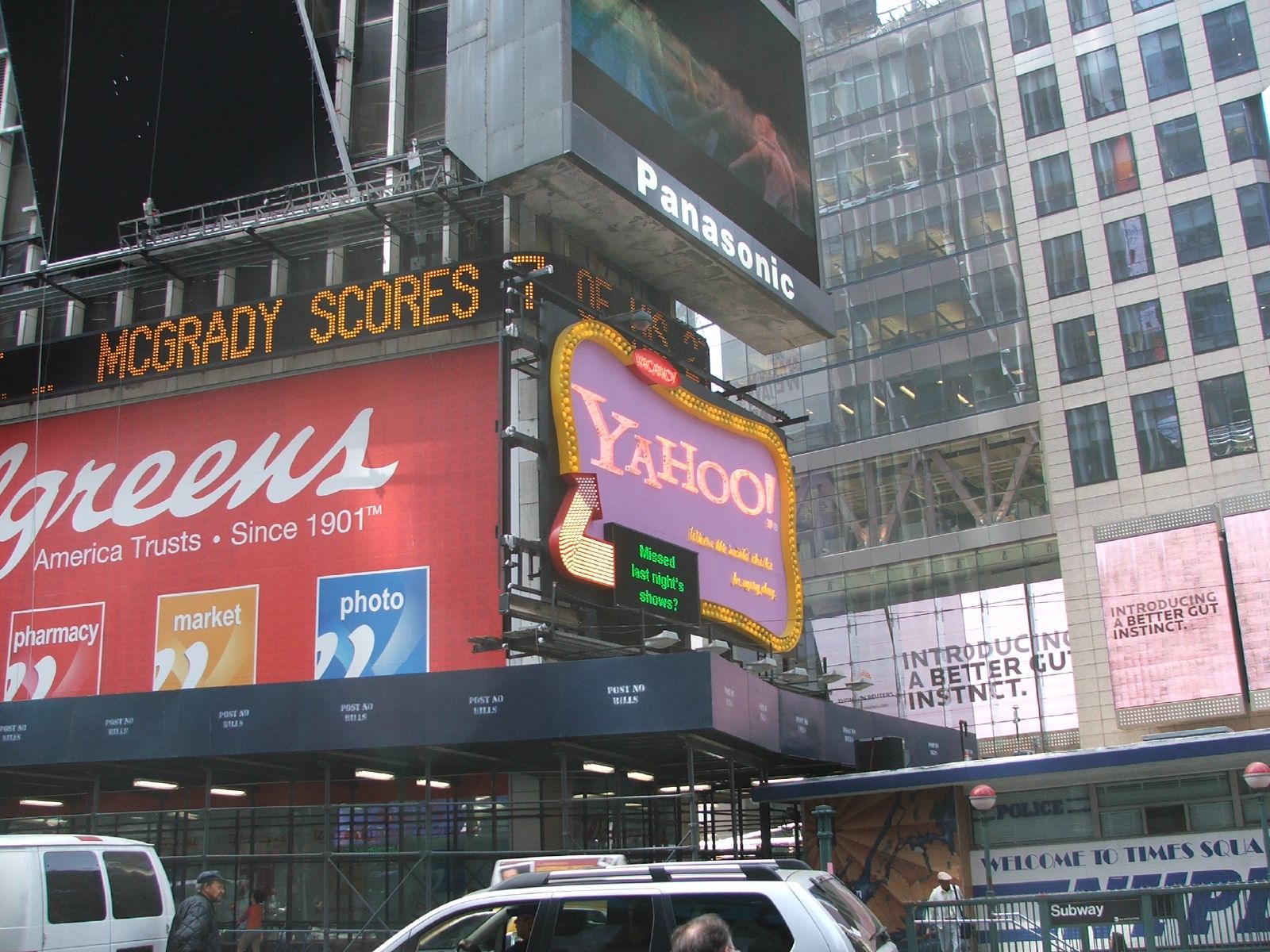This is a daytime outdoor photograph that closely resembles the bustling environment of Times Square in New York City. Prominent in the image is a large Panasonic TV mounted on the front of a building, beneath which is a nostalgic Yahoo! search engine logo, illuminated by gold lights. To the left of the Yahoo! sign is a Walgreens advertisement featuring red and white colors; only the latter part of the name, "Greens," is visible due to the partial view. Nearby, an electronic sign reads "McGrady Scores" in bright letters. To the right are the bottom sections of two brick skyscrapers adorned with various advertisements for the shops below. The street in the foreground features two white vehicles—one partially visible car and a truck—driving past. A black metal fence separates these vehicles from the row of buildings. The background includes gray office buildings with numerous windows, adding to the iconic, vibrant atmosphere with countless neon and electronic advertisements characteristic of the area.